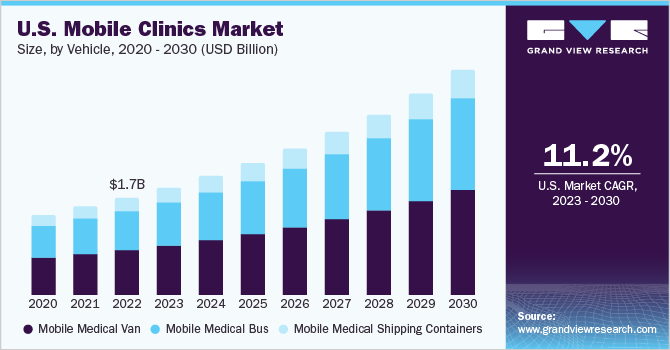This detailed bar chart, presented by Grandview Research and sourced from www.grandviewresearch.com, displays the U.S. mobile clinics market size by vehicle type from 2020 to 2030 in billions of U.S. dollars. The chart is vividly colored with bars in dark purple for mobile medical vans, turquoise blue for mobile medical buses, and light blue for mobile medical shipping containers. Each category shows a marked increase in market size over the years, highlighting a significant growth trend. Notably, in 2022, the market size reached 1.7 billion USD, and projections indicate continued growth through to 2030. An 11.2% compound annual growth rate (CAGR) from 2023 to 2030 is prominently mentioned. The chart is set against a clean white background, making the colors stand out, and the overall design is visually appealing and clearly communicates the surge in revenue for mobile medical solutions over the last decade.